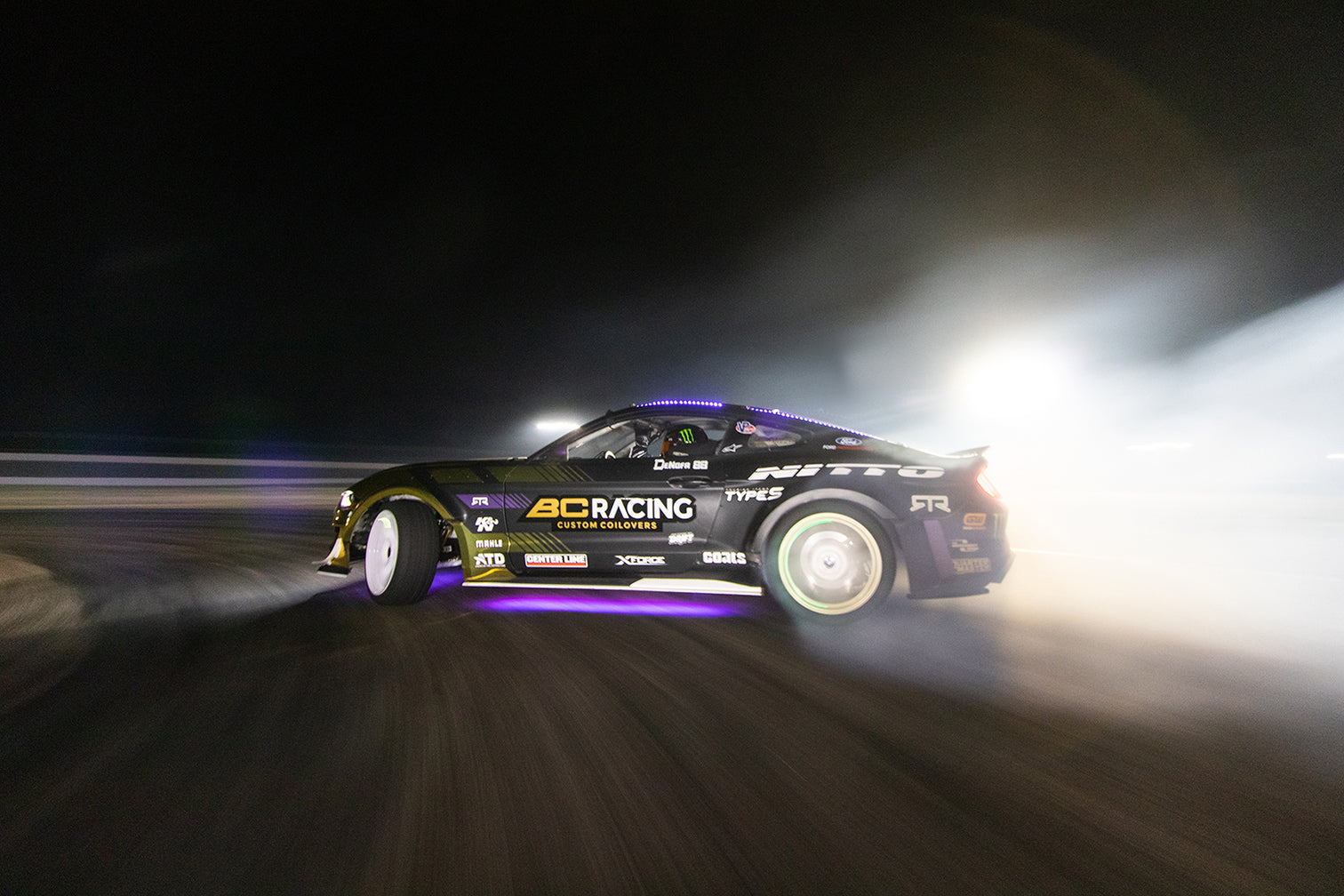In this dynamic nighttime photograph, a sleek black race car is captured mid-drift on a dimly-lit road, vividly showcasing a powerful burst of light and motion. The car is positioned centrally on the frame, against a solid black sky backdrop. Purple LED lights illuminate both the undercarriage and the roof, creating a striking visual effect. The road beneath the car features bright, cream-colored light streaks that enhance the sense of speed.

Smoke billows from the rear tires, adding to the intensity of the scene, while the car's front left tire is notably turned inward, indicating a sharp turn. Golden accents adorn this tire area, and various sponsor decals are displayed on the car, including BC Racing, Nitro Type 5, and Nitto. The driver's side door prominently features the text "B-C Racing Custom Coilovers," with additional, partially distinguishable text nearby.

The driver's helmet, black with light green stripes, is faintly visible through the blur of speed. The entire scene conveys a sense of high-speed action frozen in a moment of time, with the vehicle's motion and the surrounding blur highlighting the precision and intensity of the race.